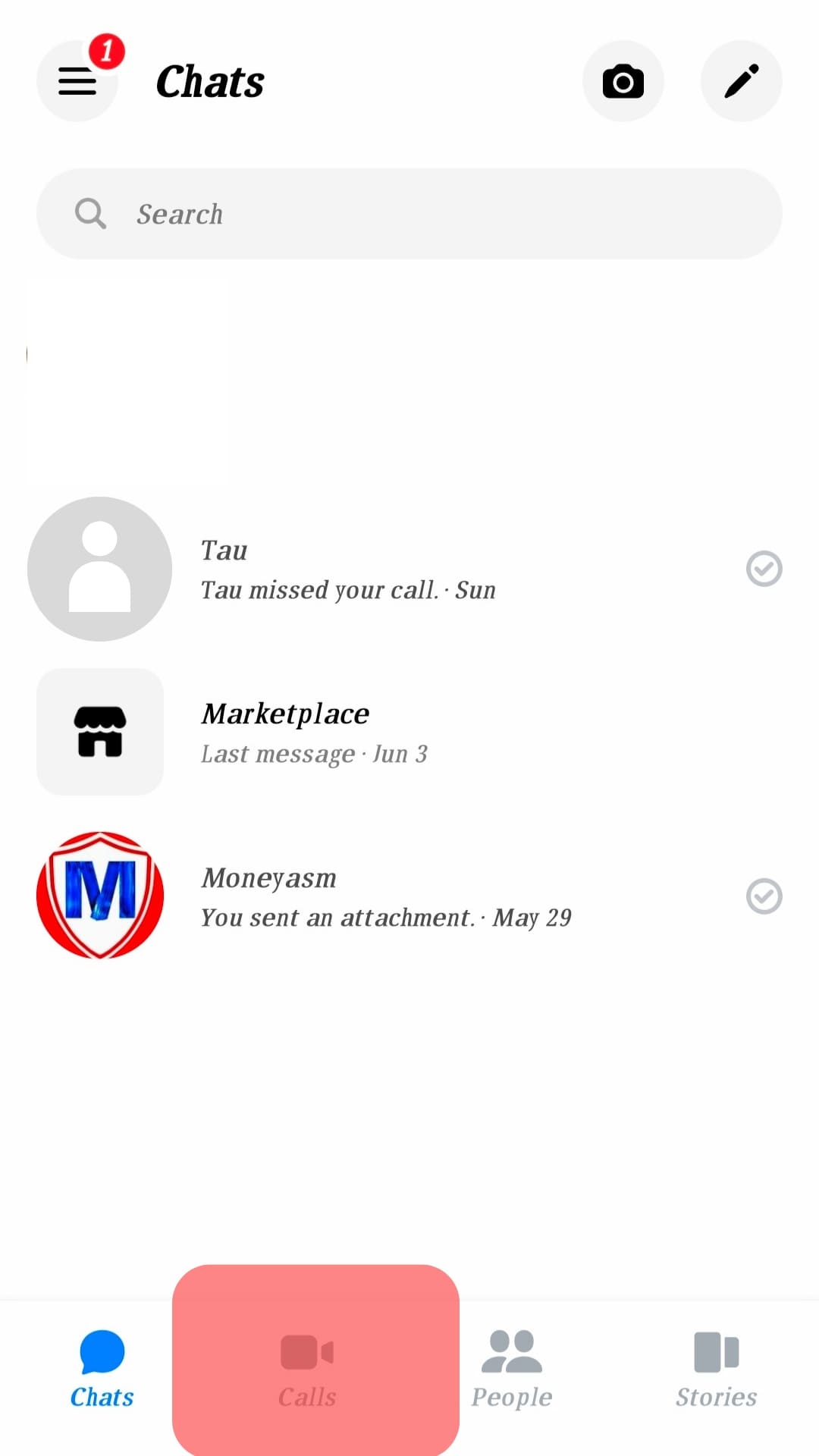The image appears to be a screenshot of a messaging application, which could potentially be either on an iPhone or an Android device—the exact platform is unclear. At the top of the screen, there's a status bar containing signal and battery indicators, followed by a notification drop-down which is not expanded, hence the notifications are not visible. Below the status bar, the interface is divided into several functional elements.

Starting from the top left, there is a "Chats" tab, with a camera icon to its right for photo or video capture and a pencil icon for composing new messages. Directly underneath these icons, a search bar labeled "Search" allows for quick access to conversations or contacts.

Under the search bar, there are three main contact entries. The first entry states "Tau missed your call on Sunday," without displaying a contact picture. The second entry, representing a marketplace feature with a logo resembling the Facebook Marketplace logo, has the information "Marketplace - last message June 3rd." The third entry is a contact named MoneyASM, which states "You sent an attachment - May 29th." MoneyASM’s logo is a distinctive blue "M" inside a white shield, which is enclosed within a red circle.

At the bottom of the screen, there is a navigation bar with four options. The "Chats" option is highlighted in blue, indicating that the user is currently on this tab. The "Calls" option appears to be unavailable, signaled by a red highlight. The "People" tab is represented by an icon of two silhouettes, and the "Stories" tab, which is presumably for short-lived content, is the last option in the navigation bar.